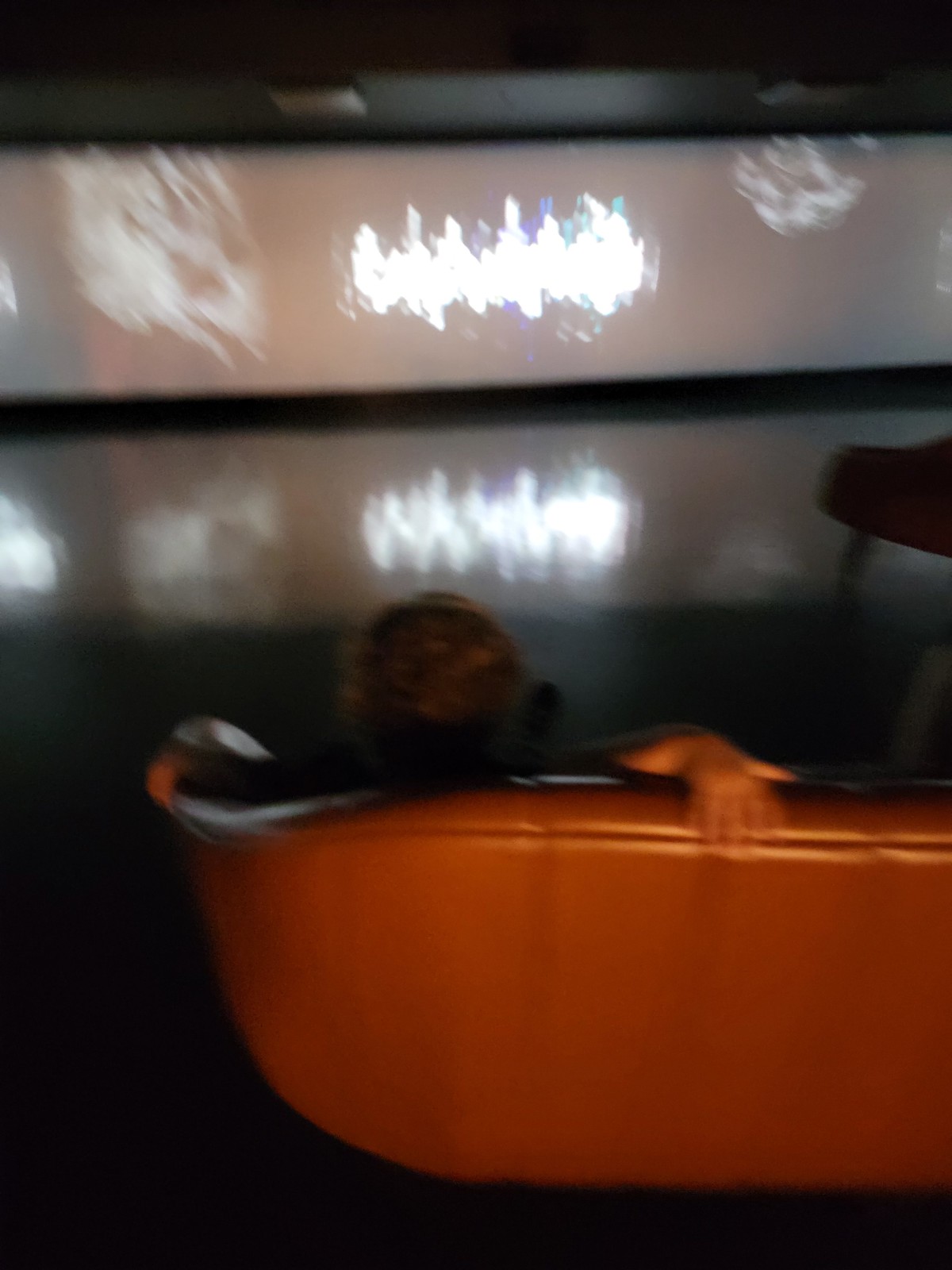This is a blurry photograph depicting a dimly lit room that resembles a home theater. Dominating the foreground is a large, leather-looking couch, described variably as brown or an orange-reddish hue. A man with light skin tone and brown curly hair, possibly wearing a headset, is casually draped over the back of the couch, with one hand resting on it. The setting is characterized by its dark ambiance, featuring a black ceiling with square white lights that are turned off. In front of the man, there's a wide screen display showing bright white, squiggly lines, accompanied by some grayish scribbles on both sides. The screen's illumination is reflected on a shiny floor below, creating a slightly less intense but similarly sized mirrored image. Additionally, a chair is visible in the background on the right side. The entire scene suggests the man might be watching something, although the image is out of focus and details are indistinct, lending the photo an overall distorted effect.